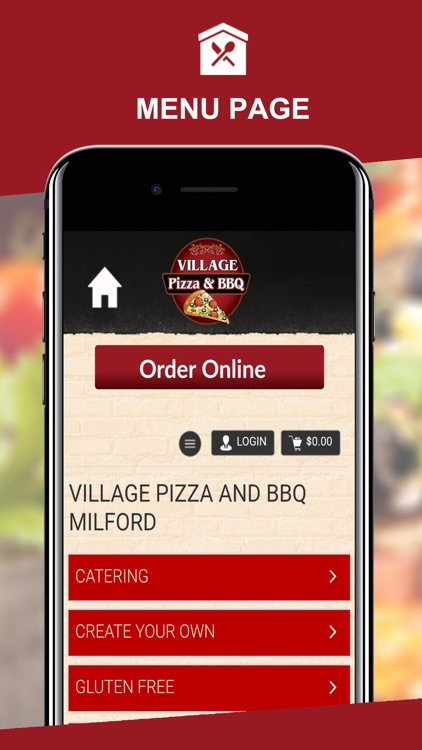This is a detailed caption for an image depicting a menu page for "Village Pizza and BBQ." The image features a brick-red colored bar running across the top with the words "MENU PAGE" boldly printed in white, capital letters. Above this bar is an icon of a house with a crossed spoon and knife, symbolizing home-cooked meals. Below the bar, there is a photo displaying a smartphone screen open to the menu page. On the smartphone, the upper left corner shows a house icon. Dominating the center of the screen is a prominent red circle with "Village Pizza and BBQ" printed inside in white text. Beneath this circle, there is an appetizing picture of a slice of pepperoni pizza. Following the image, a brick-red button labeled "ORDER ONLINE" invites users to place their orders. Directly below are two functional buttons: one for logging in and one featuring a shopping cart icon. The menu offers three options: "Catering," "Create Your Own," and "Gluten Free," each accompanied by a right-facing arrow indicating further navigation into the respective menus.